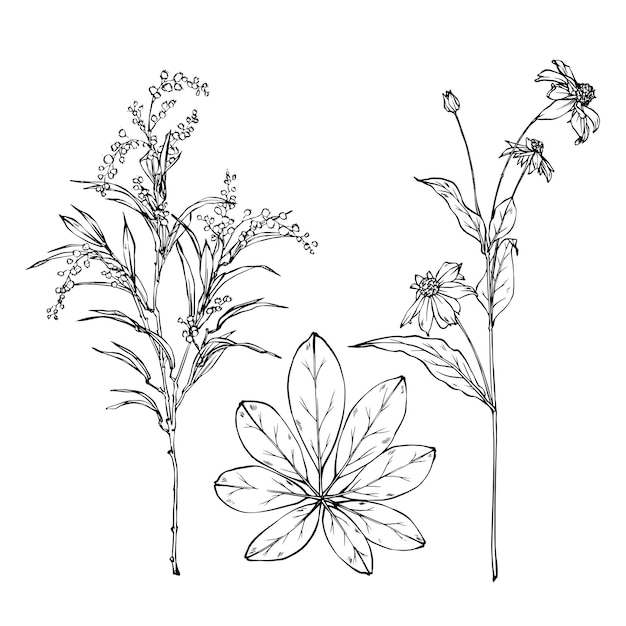A meticulously sketched black-and-white drawing depicts an intricate botanical scene. The central focus is a plant with a symmetrical arrangement of leaves. Displaying precision without shading, the plant showcases a total of eight leaves. The central leaf is the most prominent, flanked by two smaller leaves on each side. Below, three additional leaves point downward, creating a circular composition that draws the eye. 

To the left of the plant, a flowering stalk extends upward, branching into three segments, each culminating in a fully bloomed flower. On the right, another floral stem emerges, featuring three blossoms already in bloom and a fourth, poised at the top, still in bud form. The detailed linework captures the delicate structure and potential for growth of each element within the scene.